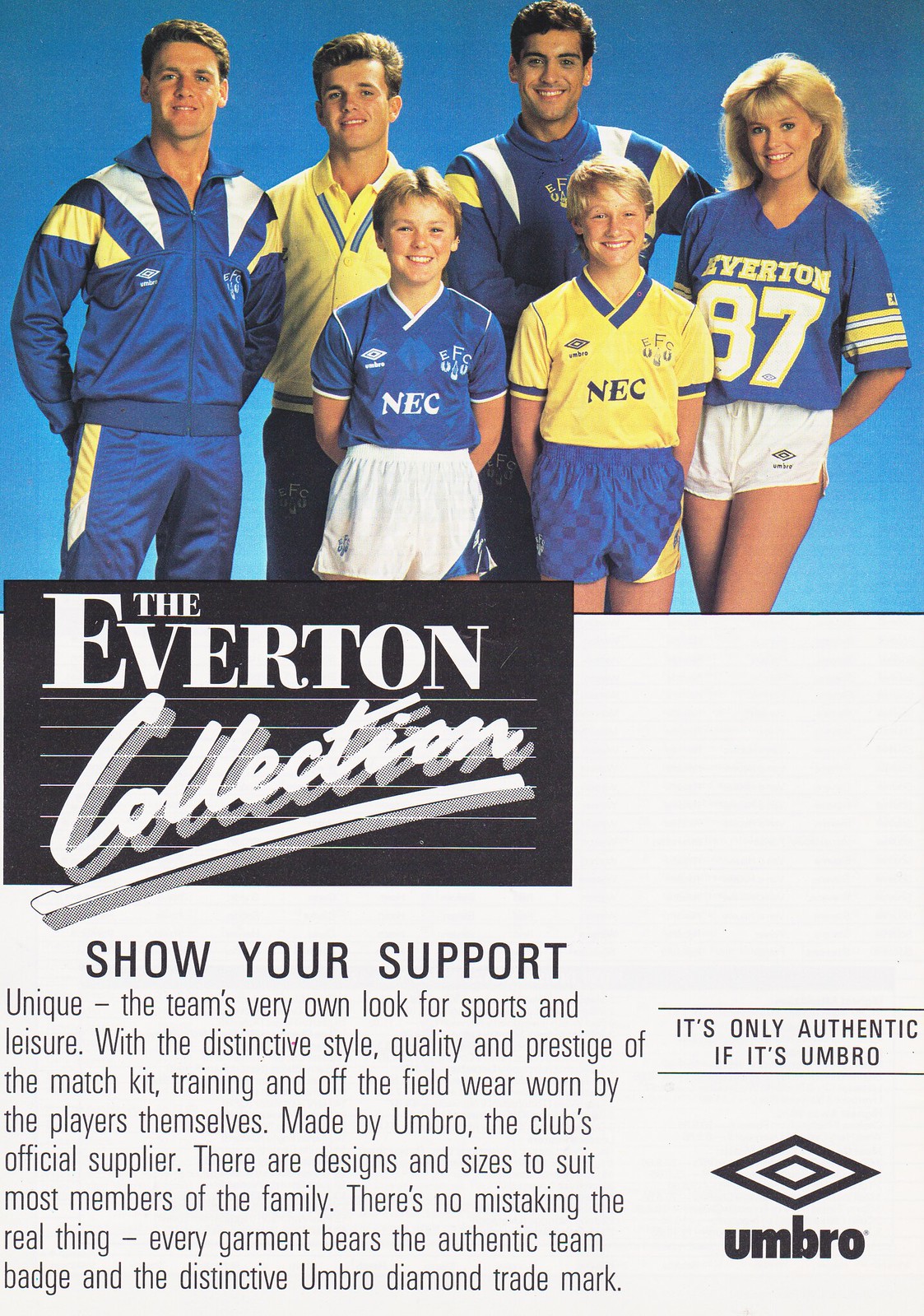This advertising photo from a sports program booklet showcases six individuals modeling the Everton Collection, made by Umbro. On the far right stands a woman with long blonde hair wearing Everton's blue and yellow V-neck jersey, numbered 87, and adorned with stripes on her left bicep. Flanking the center-front position are two boys: one in a white V-neck jersey and white shorts with blue hems, emblazoned with "NEC," and the other in a yellow NEC jersey paired with blue shorts featuring yellow stripes. In the back row, a man on the left dons a blue tracksuit accented with yellow and white shoulder stripes, while the central figure sports a yellow varsity-style jacket. Another man, positioned next to the woman, is clad in a blue and yellow sports jacket. Beneath the image, the text reads, "The Everton Collection. Show your support. Unique, the team's very own look for sports and leisure. With distinctive style, quality, and prestige of the match kit, training, and off-the-field wear, worn by the players themselves. Made by Umbro, the club's official supplier. There are designs and sizes to suit most members of the family. There's no mistaking the real thing; every garment bears the authentic team badge and the distinctive Umbro diamond trademark." The Umbro logo, a layer of diamonds, certifies authenticity.